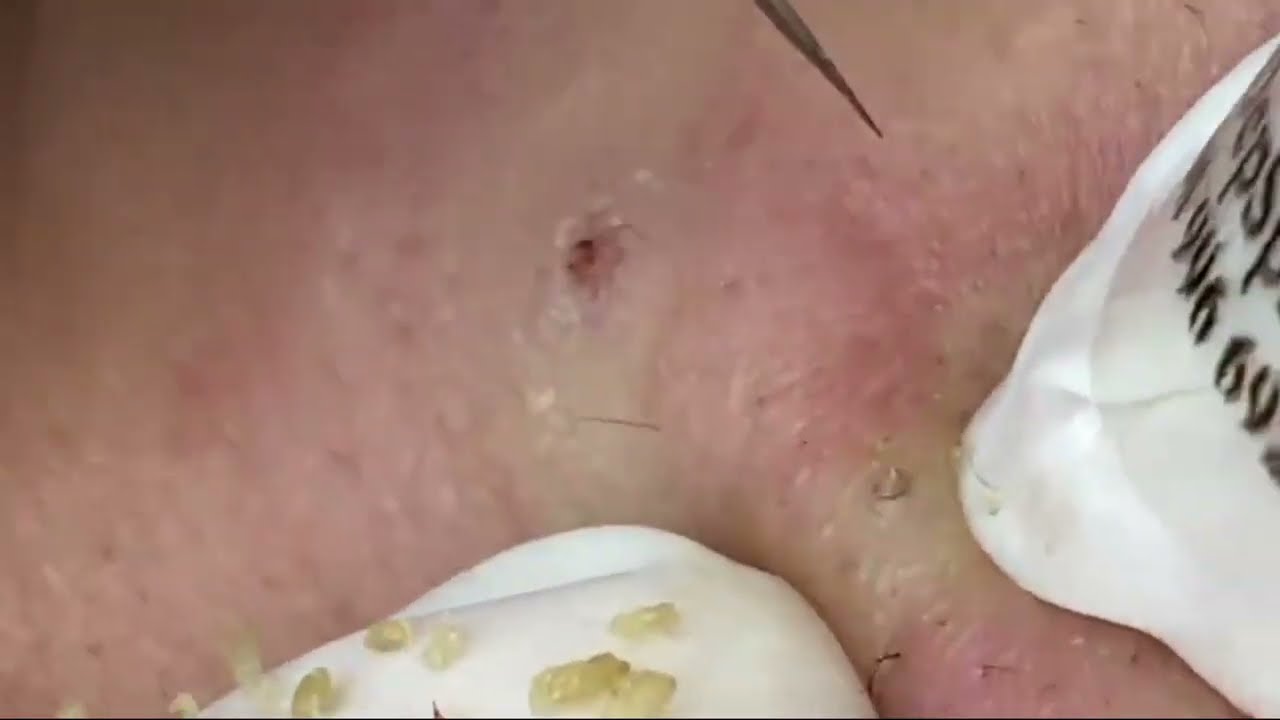The image depicts a close-up, highly magnified section of human skin, likely Caucasian, featuring a medical procedure. The horizontally rectangular, full-color photograph showcases inflamed, pink, and pale areas with visible pores and scattered hair growth. The skin appears to have openings and red spots of blood. A black pointer is positioned at the top of the image.

On the right side of the image, a white glove with partially visible black letters (EPSP) and numbers (199669 and other nines and sixes) is seen. This glove appears to be involved in squeezing yellowish-whitish pus from a pore. The left side of the image shows another white glove, smothered with the splattered goo. The procedure seems to be extracting pus from the skin, possibly using a small black instrument, leading to residue clumping on the gloved hand. Overall, it is a stark and graphic representation of a dermatological extraction process.